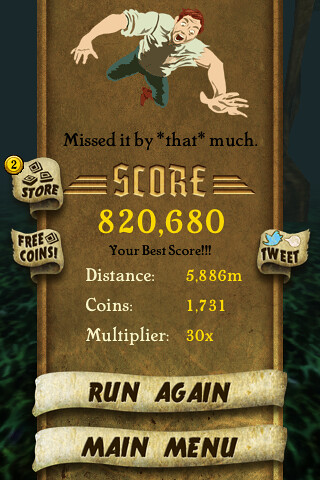The image is a detailed advertisement-like score screen, seemingly from a gambling site or mobile game. The rectangular, vertical layout features a dark green background framed by two vertical brown borders on the left and right. At the triangular top of this brown center strip, there is a cartoonish man with red hair, wide eyes, and an open mouth, appearing to be in mid-fall. He is dressed in a white shirt with rolled-up sleeves, blue pants, and brown shoes, his outstretched hand positioned over the text below him.

The text reads in black letters: "Missed it by * that * much." Directly beneath this, it lists various game statistics in a structured format, starting with "SCORE" in all caps above the numbers "820,680" highlighted in yellow. Below this, "Your Best Score" is written in black letters, followed by "Distance: 5,886 M," "Coins: 1,731," and "Multiplier: 30x" in their respective sections.

On the left border, a small circle displays the number "2," and a wavy square ribbon reads "Store," with three square boxes above labeled as "free coins." Adjacent are more navigation options, including a white banner with "Tweet" in black letters and the iconic blue Twitter bird. Similarly, on the right side of the main brown center strip, two brown banners read in all caps, "Run Again" and "Main Menu."

The overall aesthetic combines a cartoonish yet detailed depiction with a mix of hunter green, brown, yellow, and blue hues, making the screen vibrant and engaging.